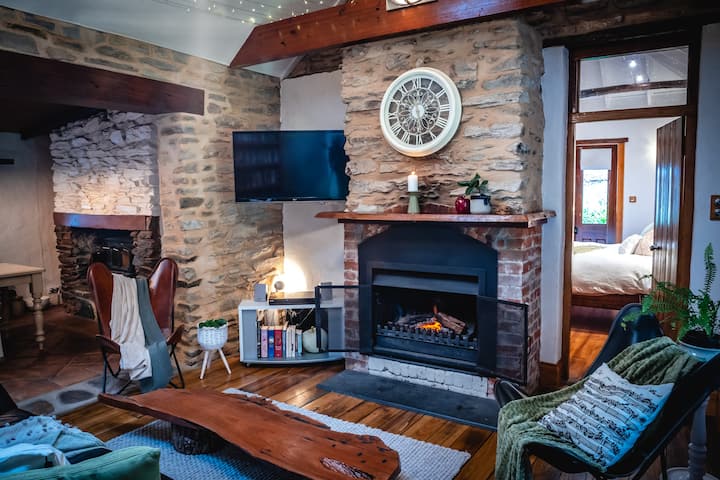This detailed photograph captures the rustic and modern interior of a cozy living room. At the center of the room is a black-framed fireplace with a soft, glowing fire, surrounded by red brick that extends into a chimney. A large, round white clock with intricate designs hangs above the fireplace. To the left, a flat-screen TV is mounted on the wall, while to the right, a different angle shows a glimpse of another brown fireplace with a stone border. The room features high-gloss wood plank flooring, with wood grain extending throughout and matching wood door casings and baseboards. In front of the fireplace sits a striking live-edge natural wood coffee table. Flanking the scene are two leather chairs, each draped with blankets, contributing to the warm and inviting ambiance. A planter adds a touch of greenery. To the right side of the room, a door opens to reveal a bedroom with a white bed. Overall, the decor highlights natural elements, blending a rustic feel with modern touches.